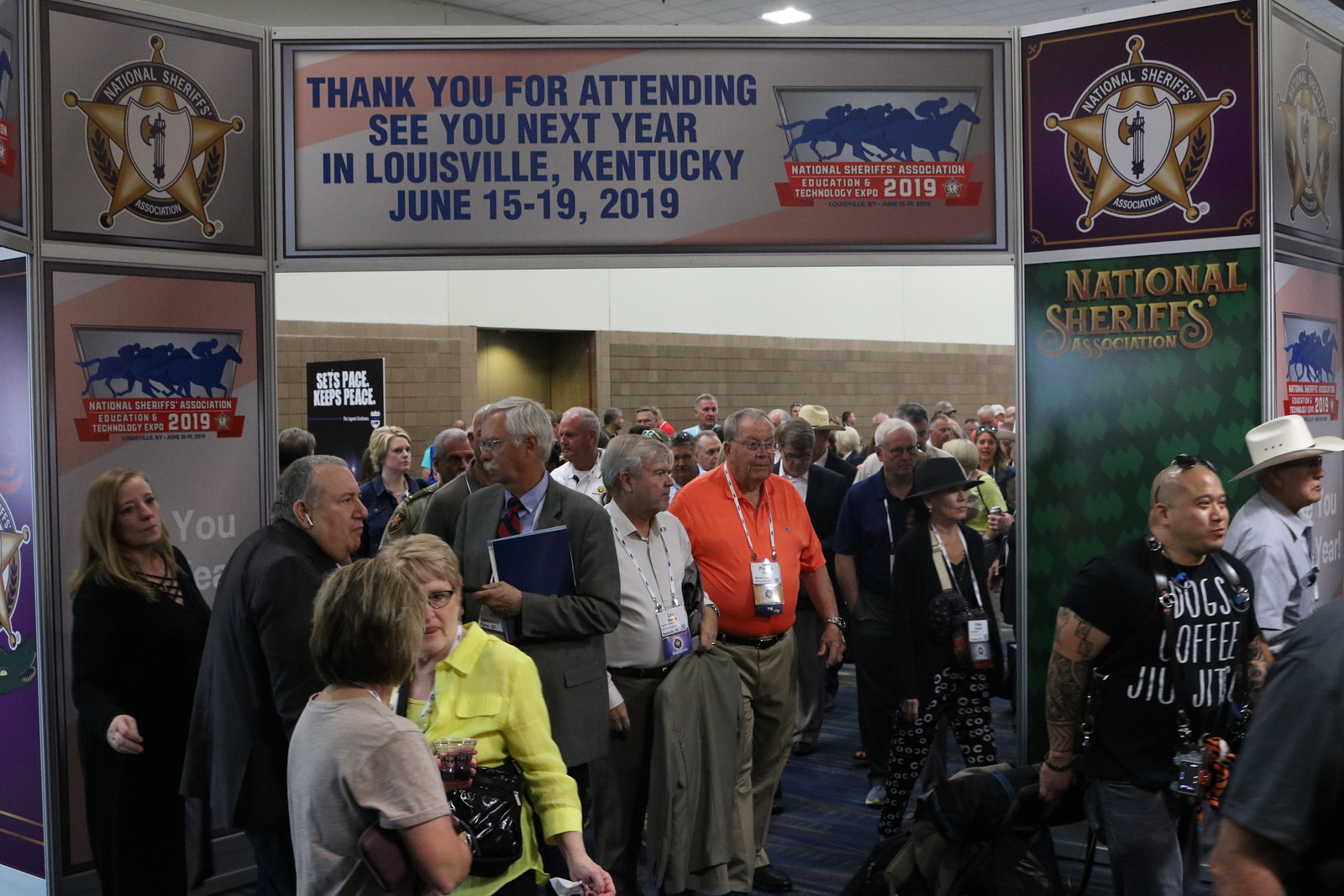The photograph captures a crowded indoor scene featuring a diverse group of predominantly older individuals, both men and women, standing and interacting under vibrant and colorful banners. The main banner prominently reads, "Thank you for participating. See you next year in Louisville, Kentucky, June 15-19, 2019," and is adorned with vivid colors like red, blue, and purple with white text. The setting is associated with the National Sheriff's Association's annual conference, evidenced by multiple logos displayed throughout, including golden sheriff's deputy badges and circular emblems featuring the text "National Sheriff's Association." The banners, positioned on the back walls and above head level, enhance the festive atmosphere. Attendees wear a variety of clothing colors such as black, white, gray, red, and yellow. The detailed decoration includes imagery of men riding horses, further emphasizing the event's connection to the National Sheriff's Association. Despite some elements suggesting a horse racing theme, the setting is clearly marked by its focus on the annual conference and gathering of law enforcement professionals.